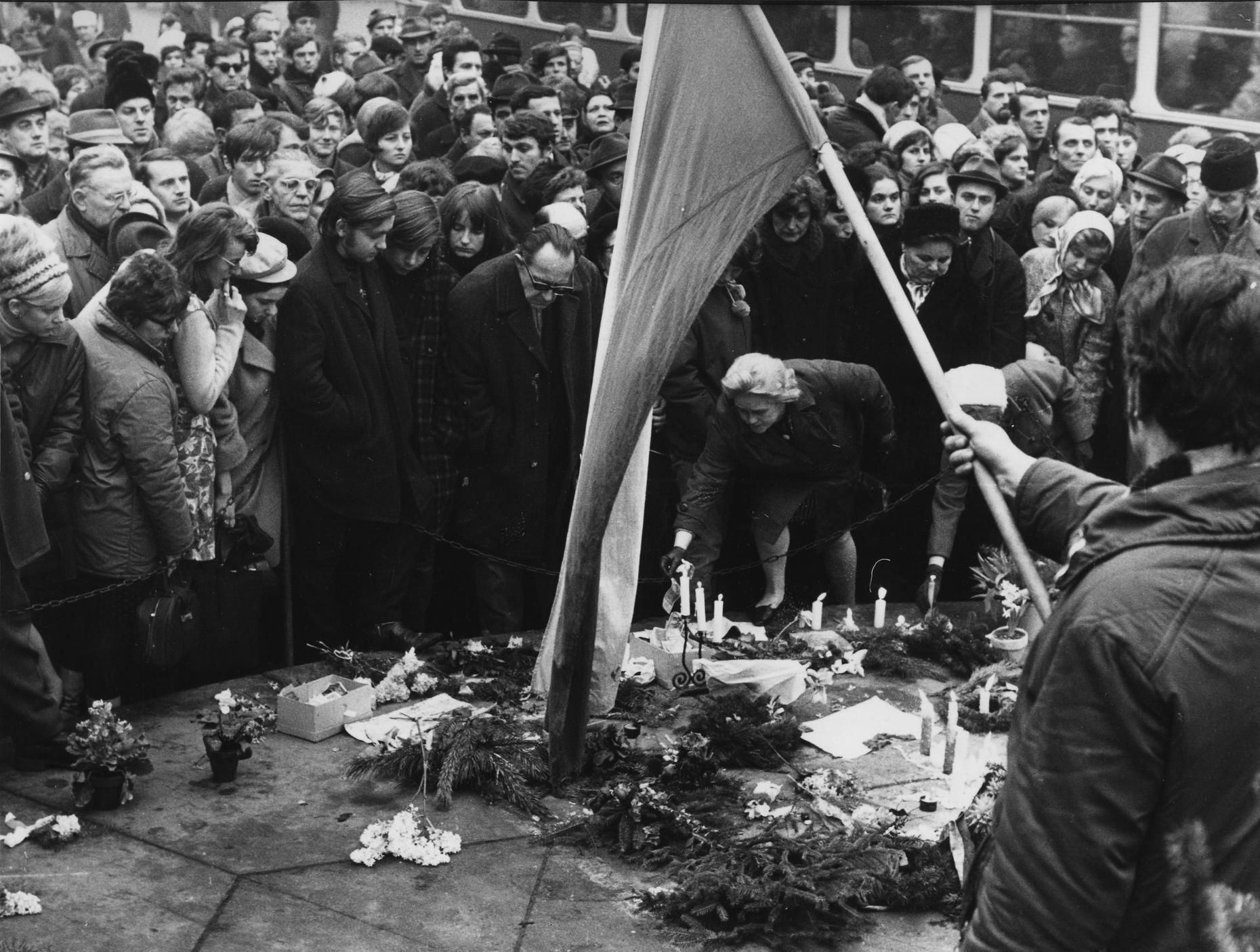This black and white photograph captures a somber gathering at a memorial or a candlelight vigil, likely from the 50s or 60s based on the style of clothing and headgear, including long black coats, sunglasses, and fedoras. The focal point of the image is a memorial surrounded by numerous plants and candles, creating a concentrated display at its center on what appears to be a hexagonal and triangular cobblestone street. The area is roped off with a metal chain, signifying its importance. 

On the right side of the memorial, a woman with curly hair, dressed in a long gown, is seen bending down to place a candle among the others. Meanwhile, towards the back, another woman with short hair holds a tall flagpole, the flag draping towards the center, yet its design remains indiscernible. 

A multitude of individuals, dressed warmly in winter coats and hats, are gathered, some gazing solemnly at the memorial, others looking towards the flag or at the woman placing the candle. Expressions are serious and contemplative, reflecting the gravity of the occasion. Cards or notes accompany the numerous flowers and candles, signaling personal tributes from attendees. In the background, a vehicle, possibly a train or bus, is visible with people inside, adding to the crowded scene. The overall tone captured is one of quiet reverence and collective mourning.